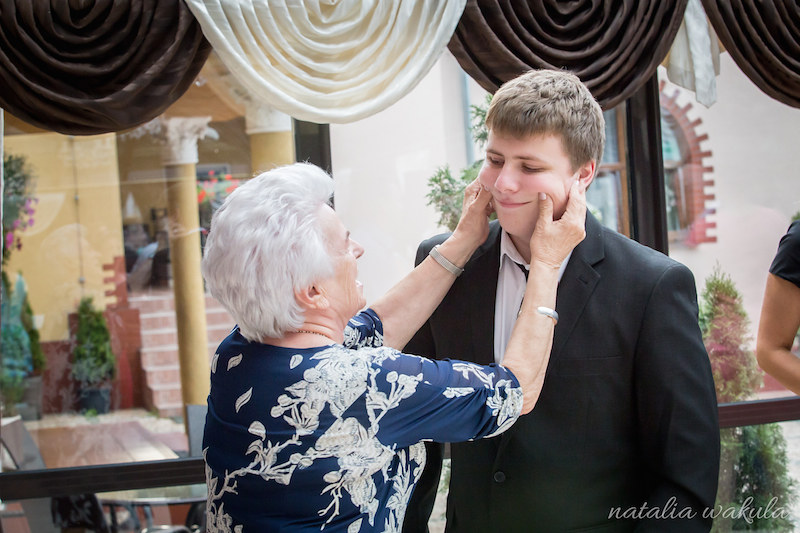In this outdoor celebration photo, an older woman with elegant gray hair and a blue and white floral dress is smiling warmly while pinching the cheeks of a younger man, who is also smiling back at her. The man, likely her grandson, is dressed in a suit jacket with a white shirt and an open, loosened tie, suggesting a semi-formal occasion. The backdrop features a picturesque, formal setting with stone pillars, decorative draperies, and steps leading to what appears to be a reception area. A table and chairs can be seen, enhancing the festive ambiance. Additionally, there is a partial view of another individual standing to their right. The photograph, taken in the daytime, bears the digital signature "Natalia Wakula" in the bottom right corner.